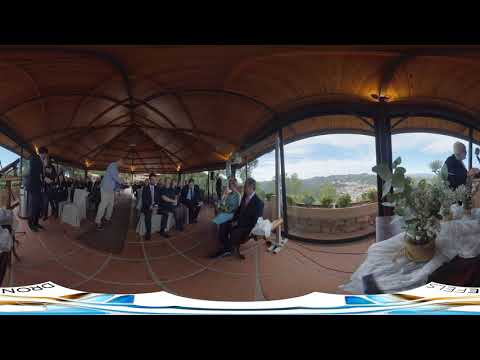This photograph captures an indoor-outdoor pavilion with a rustic, orange-brown teak wood roof and a red-tiled floor with gray grouting, arranged in a checkered pattern. The scene appears to be an elegant, formal event, likely a wedding ceremony. Guests are dressed in dark suits, ties, and formal dresses. In the center, there is a long aisle, suggestive of an impending procession, possibly for a bride and groom. The left side of the pavilion has people standing, while the right side features decorated tables with white and green flowers. Various attendees, some seated and others standing, are engaged in quiet conversation. In the background, through open sides of the gazebo, a picturesque landscape of green trees, mountains, and a blue sky dotted with white clouds can be seen, enhancing the serene and joyous atmosphere of the celebration.